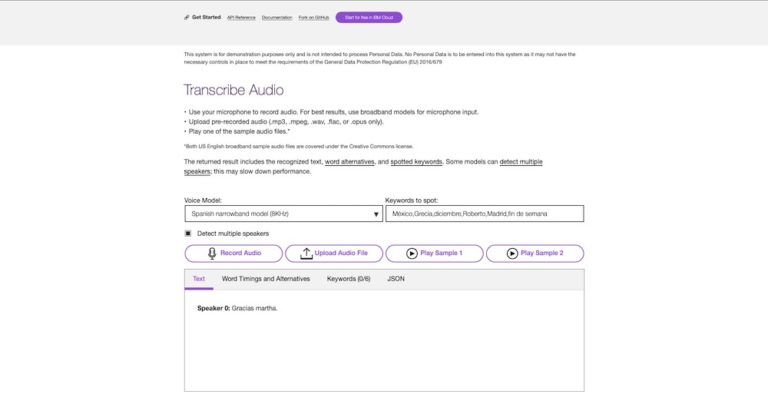Screenshot Description:

The screenshot depicts a web page with a predominantly white background. At the very top of the page, there are four menu options, although the exact text of these options is not readable due to small font size. One of the menu options is highlighted with a purple oval. Just below the menu, there is some text, but only the phrase "transcribe audio" is discernible.

Further down the page, there are buttons also highlighted in purple circles. These buttons are labeled "Record Audio," "Upload Audio File," "Play Sample 1," and "Play Sample 2." Below these buttons, there is a coding section with two input boxes. The first box has the label "Voice Model," and the second is labeled "Keywords to Spot." The rest of the text on the page is too small to read clearly. The layout is predominantly white with accented elements in purple, including text and ovals.